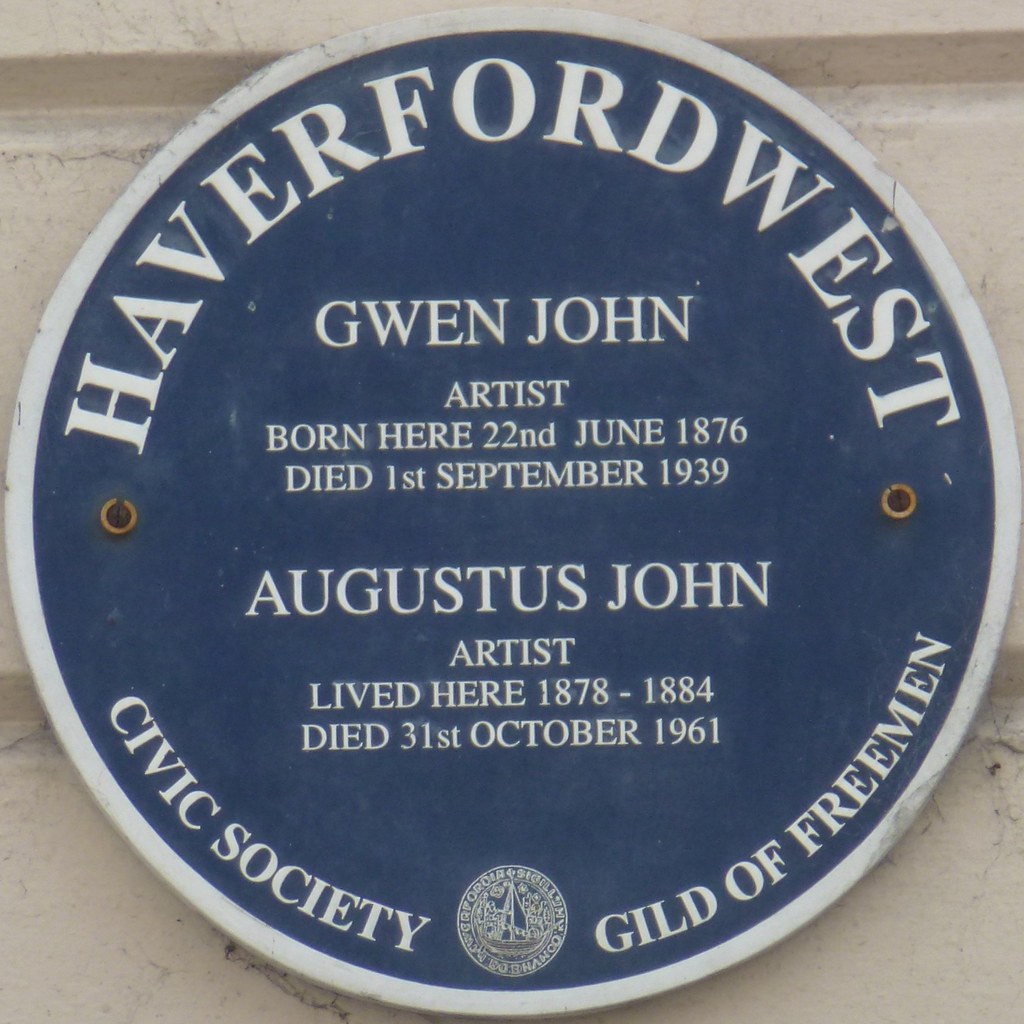A vivid photograph captures a round plaque affixed to a white brick wall, held in place by two copper-colored bolts. The plaque has a dark blue interior with crisp white lettering, bordered by a white rim. Across the top, it prominently reads "Haverfordwest." Below, detailed inscriptions honor two artists: "Gwen John, Artist, born here 22nd June 1876, died 1st September 1939," followed by "Augustus John, Artist, lived here 1878 to 1884, died 31st October 1961." At the bottom, the plaque features the text "Civic Society Guild of Freeman," with a detailed white logo or seal centered beneath this line. The plaque commemorates the birthplace and residence of these notable artists, signifying their historical significance to the location.